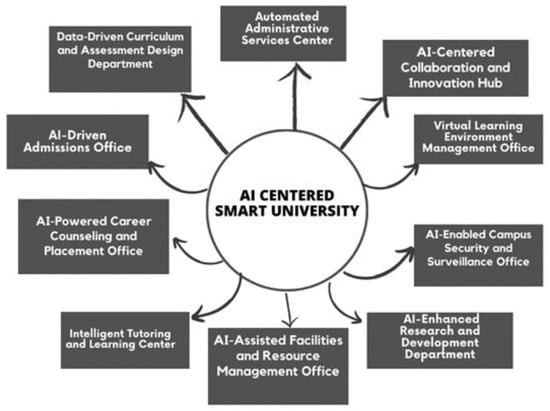The infographic illustrates an AI-Centered Smart University and is set on a white background. At its core, there is a central white circle with dark grey text reading "AI-Centered Smart University." Encircling this central node are ten arrows radiating outwards, each leading to a rectangular, dark charcoal grey box. These boxes, labeled in white text, represent different departments within the university. Starting from the top and moving clockwise, the departments are: Automated Administrative Services Center, AI-Centered Collaboration and Innovation Hub, Virtual Learning Environment Management Office, AI-Enabled Campus Security and Surveillance Office, AI-Enhanced Research and Development Department, AI-Assisted Facilities and Resource Management Office, Intelligent Tutoring and Learning Center, AI-Powered Career Counseling and Placement Office, AI-Driven Admissions Office, and finally, Data-Driven Curriculum and Assessment Design Department. This flowchart visually emphasizes the integration of AI in handling various administrative and educational functions, underscoring the smart, automated operations of the university.